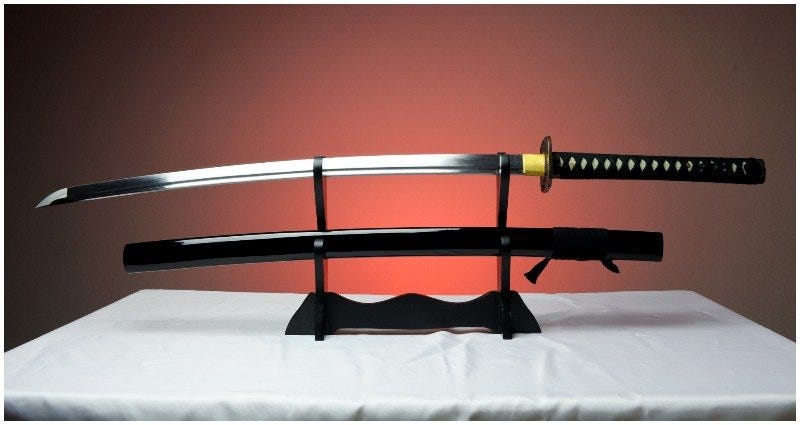This digital image captures a meticulously displayed samurai sword on a white tablecloth-draped table. The sword, with a long, sharp steel blade with a hint of black hue at the beginning and end due to lighting, rests on a dark wooden stand. This stand has two levels, with the sword on the top and the equally long, all-black sheath with a dangling ornament on the lower tier. The handle of the sword is black, adorned with evenly spaced white diamonds that slightly wear towards the end, signifying usage. A yellow ribbon accents the handle just before the blade guard. The background features a gradient, darkening from the reddish-orange center to near-black edges, creating a highlighted orb-like effect that dramatically emphasizes the weapon, almost resembling a setting sun.